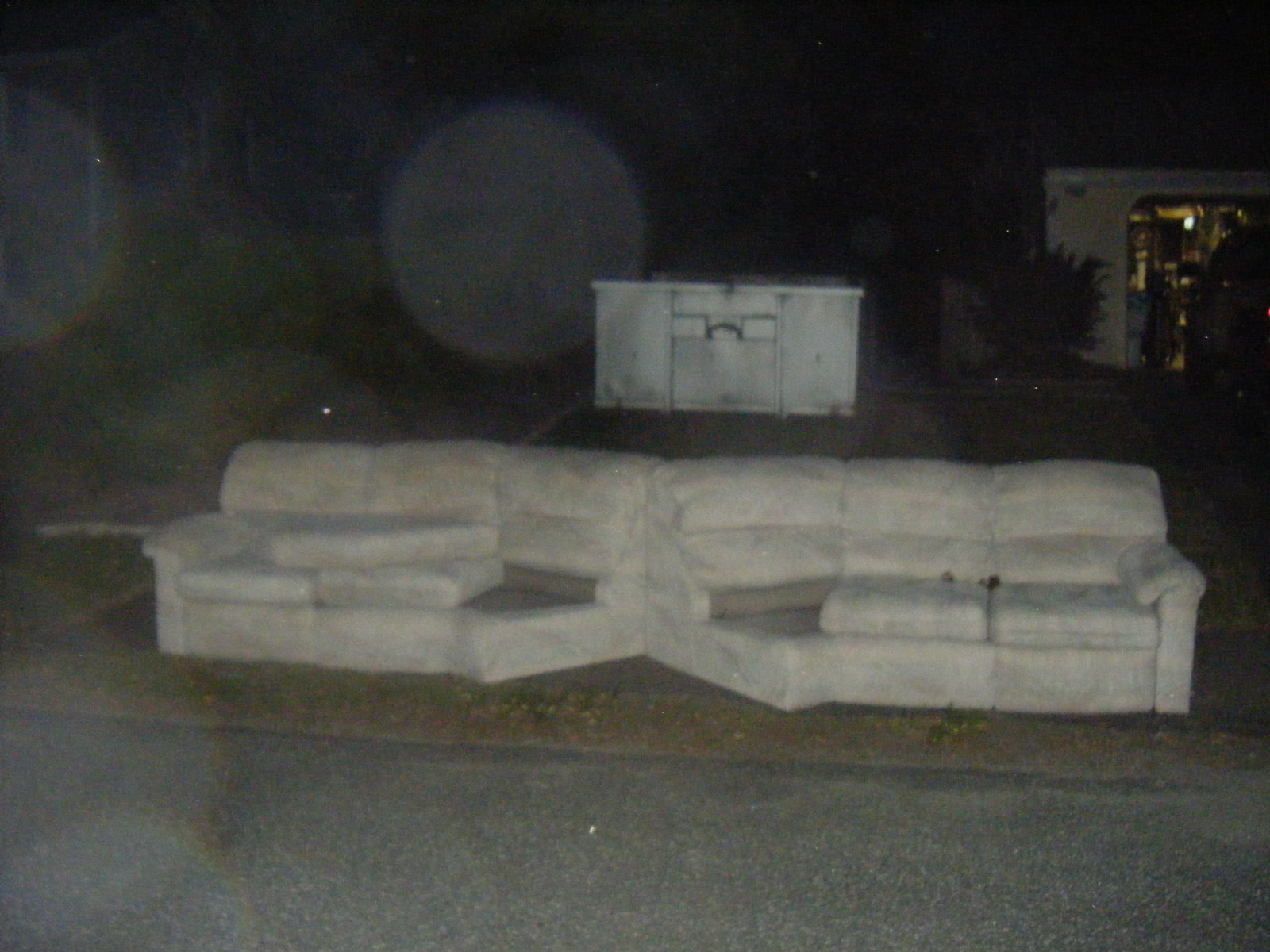This image captures a very grainy and blurry night scene featuring a dirty, off-white/lights gray sectional couch in disarray. The sectional, meant to form a corner, has been spread out into a straight line with its two sections now facing opposite directions—one to the right and one to the left. The cushions are noticeably filthy and there are square cushions stacked on top of each other, creating a triangular shape. A cushion appears to be missing from the three-seater portion on the right. This couch is set outside, on the side of a street with an asphalt road in front. In the background, there is a large silver-gray container, possibly a dumpster, and to the right, an opening of a building resembling a shop or house garage, from which a faint yellow-orange light is emanating. Some spots and circles caused by lens flares and the general graininess of the photo are also noticeable, contributing to its fuzzy and obscure quality.